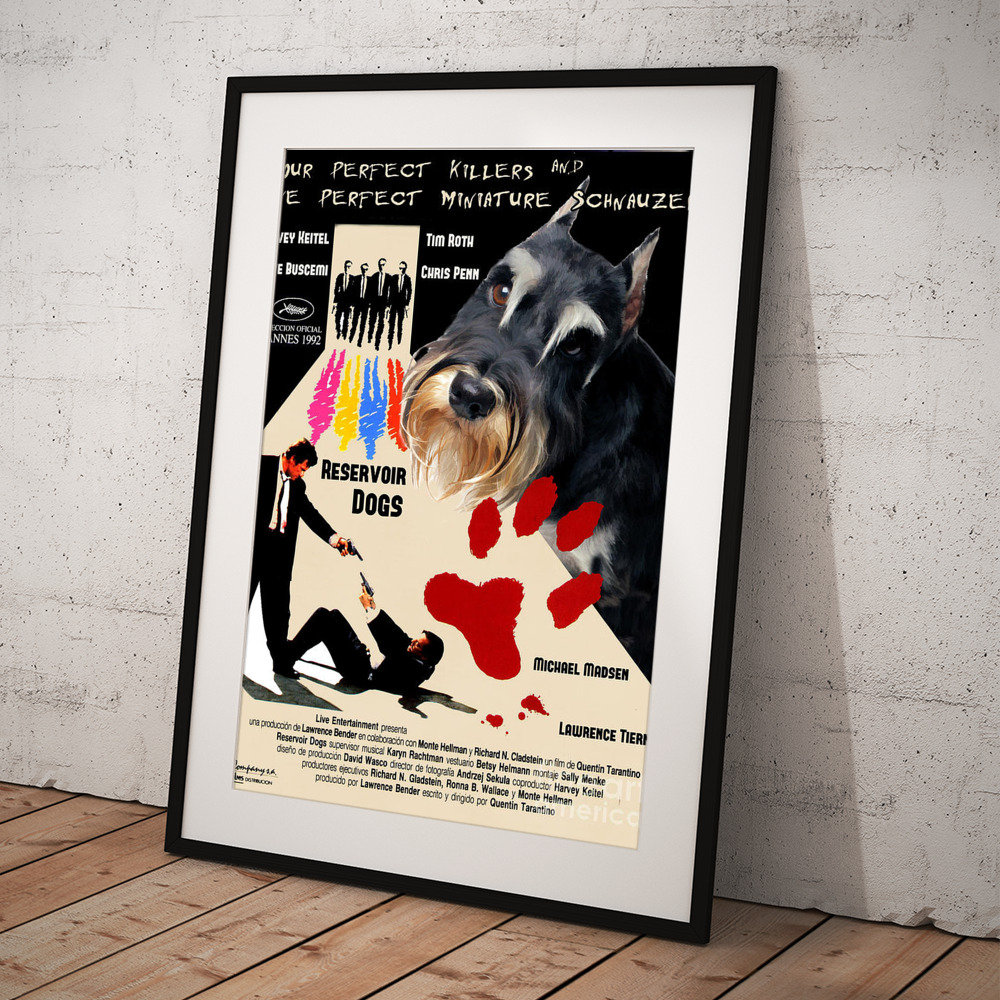The framed poster, measuring approximately three feet tall, is presented in a thin black frame with a thick white matting about an inch wide. It rests against a textured, gray-painted cinder block wall, standing on a newly installed wooden floor that lacks polish or shine. The poster, advertising the film "Reservoir Dogs," features four men clad in black suits, each casting a uniquely colored shadow in pink, yellow, blue, and red. In a playful touch, the poster includes a miniature schnauzer head and a red-colored paw print. The details of the film’s cast, including Michael Madsen, Tim Roth, Chris Penn, Steve Buscemi, and Harvey Keitel, are prominently displayed. The foreground depicts two characters in a dramatic standoff, guns drawn at each other, surrounded by the vibrant colors and the unique artistic elements, making it a visually striking piece.